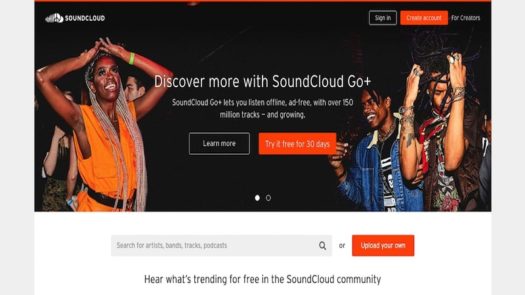This image features the homepage of SoundCloud, a prominent music streaming platform. In the top right corner, there are options to sign in or create an account, the latter highlighted in orange to attract creators. Below, a vibrant scene depicts people dancing joyfully to music, reflecting the lively spirit of SoundCloud. 

The centerpiece text promotes SoundCloud Go+, an enhanced version of the service. It reads, "Discover more with SoundCloud Go+," followed by details about its benefits: offline listening, ad-free experience, and access to over 150 million tracks with more being added continually. Users are encouraged to learn more and try it free for 30 days. Additionally, the webpage invites users to search for artists, bands, tracks, and podcasts, or to upload their own content. It also encourages users to explore trending content within the SoundCloud community for free.

The color palette of the image includes a mix of black for the background, with vibrant accents of orange, blue, red, and white, creating a dynamic and engaging visual experience.